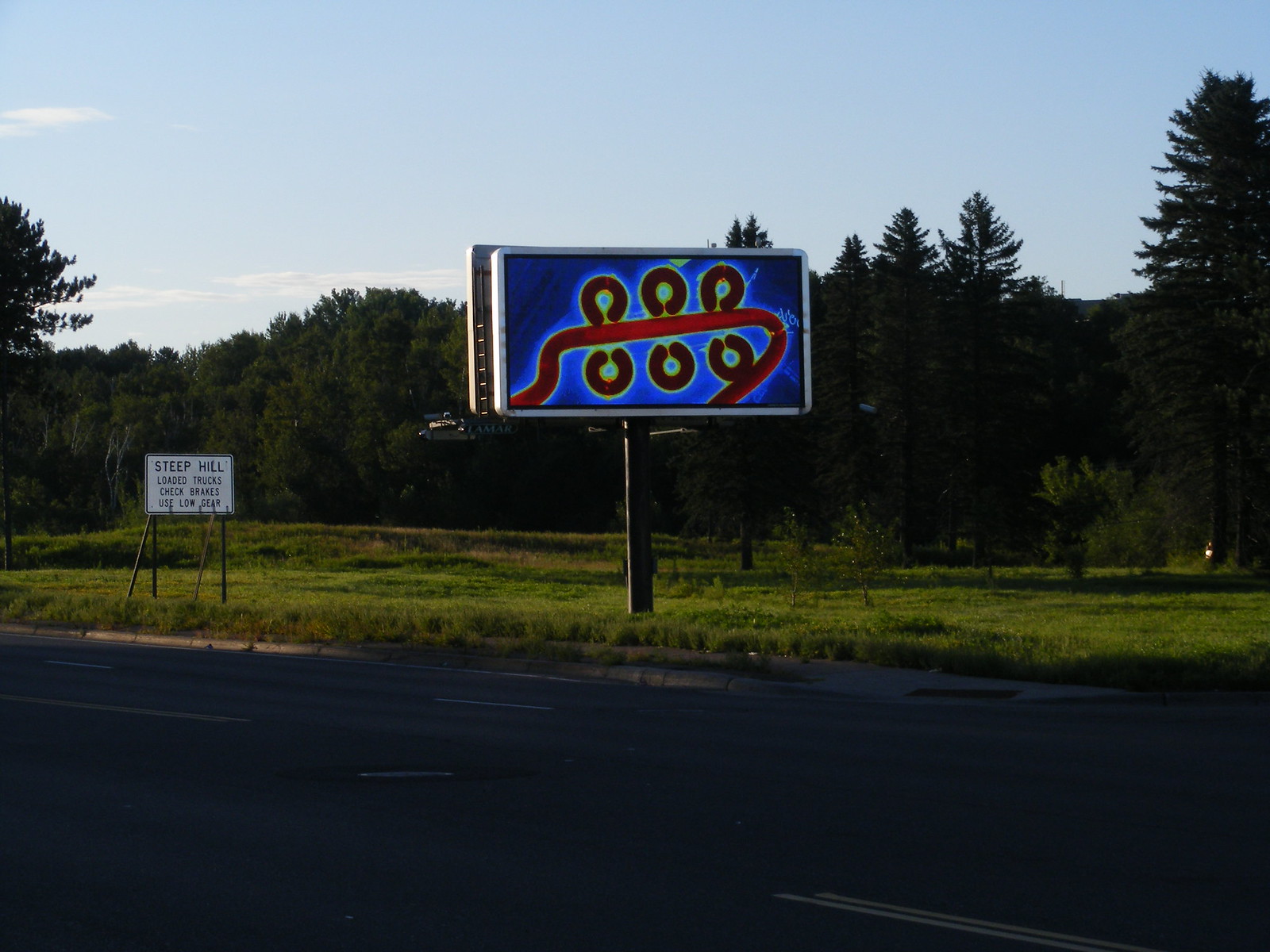This photograph showcases an unusual and vibrant billboard situated along a stretch of highway bordered by lush green grass. The billboard stands out with its unique design, featuring a navy blue background that brightens to cobalt blue in the center. Adorned with six nearly circular red squiggles, each outlined in yellow or neon green, the billboard's layout includes three of these shapes arranged in a row at the top and three at the bottom, with a large red squiggle weaving upwards between them and back down to the corner, resembling a worm-like pattern. To the left of the billboard is a white road sign warning, "Steep Hill, Loaded Trucks, Check Brakes, Use Low Gear." Set against a backdrop of various trees, including evergreens and leafy varieties, the scene is framed under a light blue sky with a few clouds. The surroundings, characterized by a flattish black asphalt road and a hill in the distance, present a more muted color palette, contrasting sharply with the vibrant hues of the billboard.